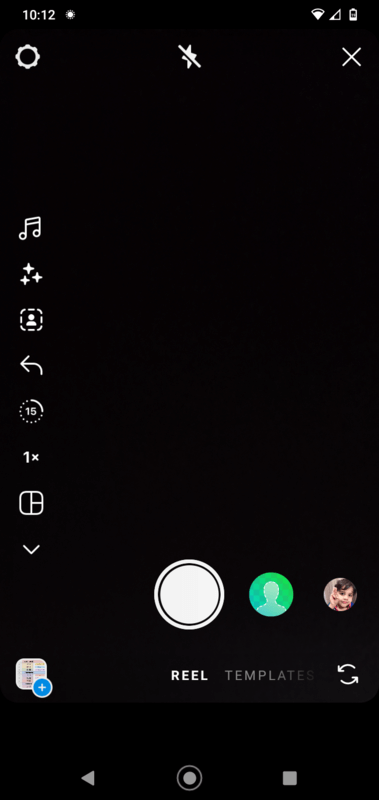**Caption:**

A detailed screenshot from a social media app, likely Instagram or TikTok, displaying the interface for recording a reel. The screen has a black background. 

- **Top Section:** 
  - Top Left: The current time and a red record symbol indicating an active recording.
  - Top Right: Icons for Wi-Fi signal, data signal, and battery life.

- **Below the Top Bar:**
  - A settings icon, a flash symbol, and an 'X' to close the app.

- **Left Side Vertical Menu (from top to mid-screen):**
  - A music note icon, a three-star icon, a portrait icon with a dashed outline, a reply button, a 15-second timer, a '1x' zoom marker, a collage icon, and a downward-pointing arrow.

- **Lower Left Section:**
  - An image gallery with a plus symbol indicating previous pictures.

- **Center to Lower Section:**
  - The main record button, accompanied by a green circle with a portrait outline and a small image of a boy.

- **Labels Underneath the Main Icons:**
  - "Reel," "Template," and a refresh icon represented by two arrows pointing in opposite directions.

- **Bottom Strip of the Screen:**
  - A triangle for the back button, a close button, and a stop button for recording.